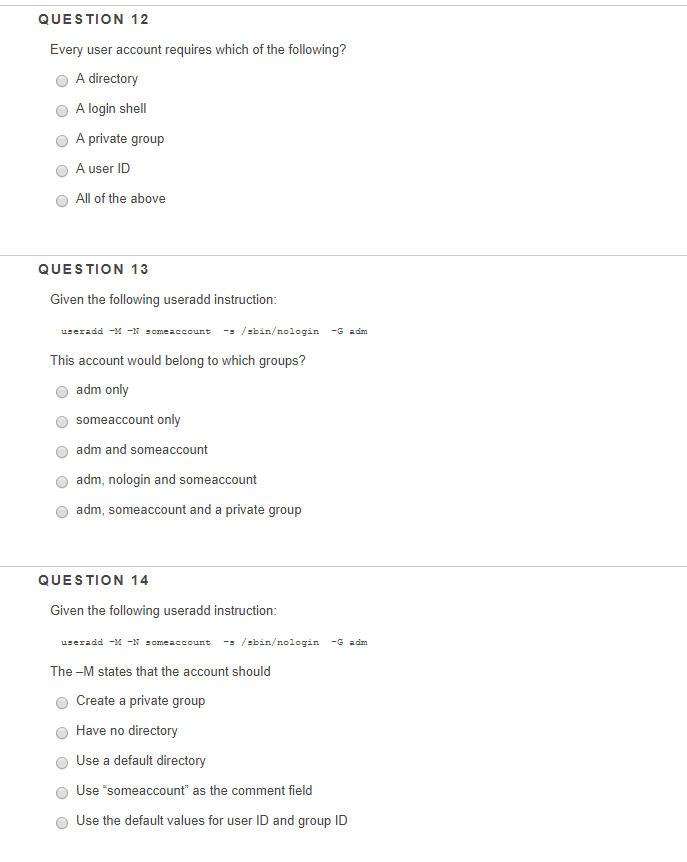The image depicts a screenshot of a computer screen showing an online quiz related to user account management and computer coding. The current question is number 12, prominently displayed in bold numerals: "12." The question reads, "Every user account requires which of the following?" Below this, there are five selectable options: "A directory," "A login shell," "A private group," "A user ID," and "All the above." Each option is accompanied by a gray button, indicating that one must be selected.

A gray line separates the current question from the next, which is question number 13. This next question asks, "Given the following 'useradd' instruction, this account would belong to which groups?" The choices provided are "Admin only," "Some account only," "Admin and some account," "Admin no login and some account," and "Admin, some account, and a private group."

Further down is question number 14, which states, "Given the following 'useradd' instruction," followed by computer code. The question focuses on the implications of the "-m" option in the 'useradd' command. The possible answers are "Create a private group," "Have no directory," "Have a default directory," "Use some account as the comment field," and "Use the default values for user ID and group ID."

Overall, the quiz is designed to assess knowledge of computer systems and user account configurations.